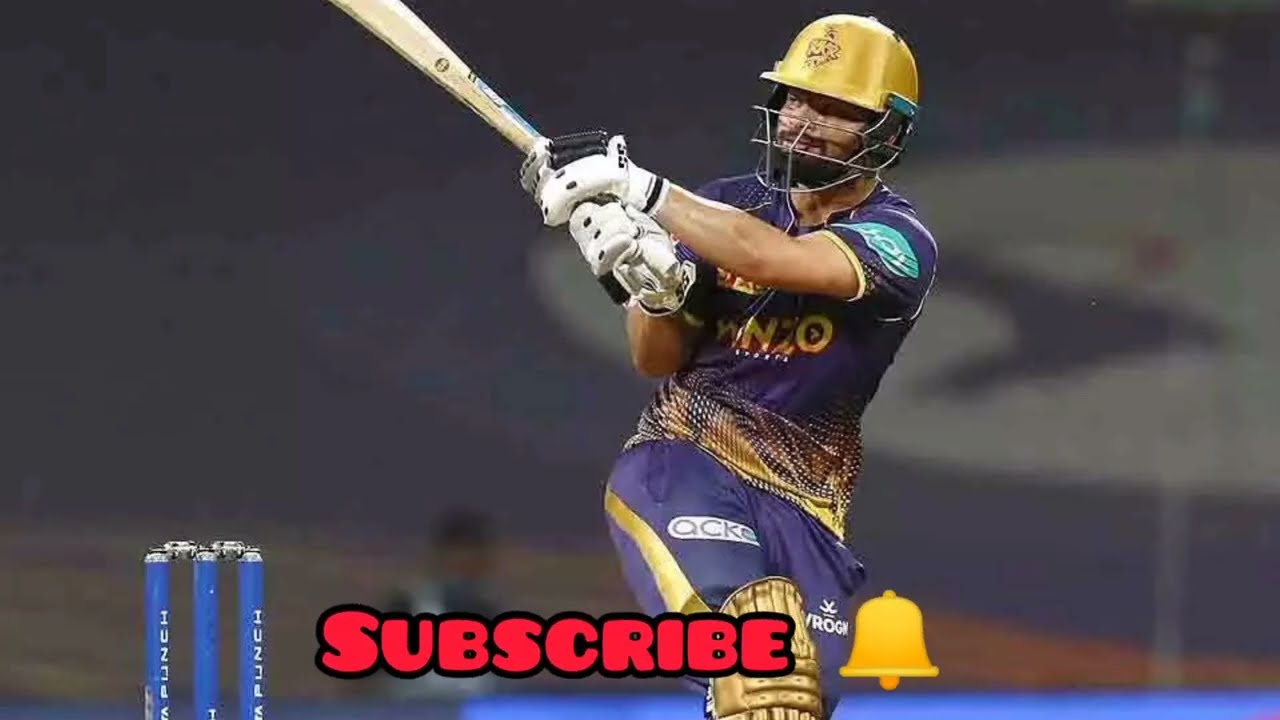The image captures a cricket player in mid-swing, holding a light brown cricket bat with both hands, his thick white gloves accented with black. The bat is slightly cropped out at the top left of the image. The cricketer is donned in a purple jersey adorned with various logos; a teal one on his shoulder, a yellow-font logo in the middle, and a dotted pattern with yellow accents lower on the jersey. He gazes towards the top left of the image, and his golden helmet, reminiscent of an NFL helmet, features thin steel bars for protection. His brown skin and beard are visible beneath the helmet. Lower in the frame, his shorts, also in purple with a gold stripe on one leg, are padded and sport additional logos—a circular white logo and another white logo on different parts of the shorts. At the very bottom center, the red, bubbly-font text reads "Subscribe" next to a yellow bell emoji. The background is blurred, showcasing indistinct shapes and colors but primarily focusing on the player. On the bottom left, three vertically-lined blue cylinders can be seen.